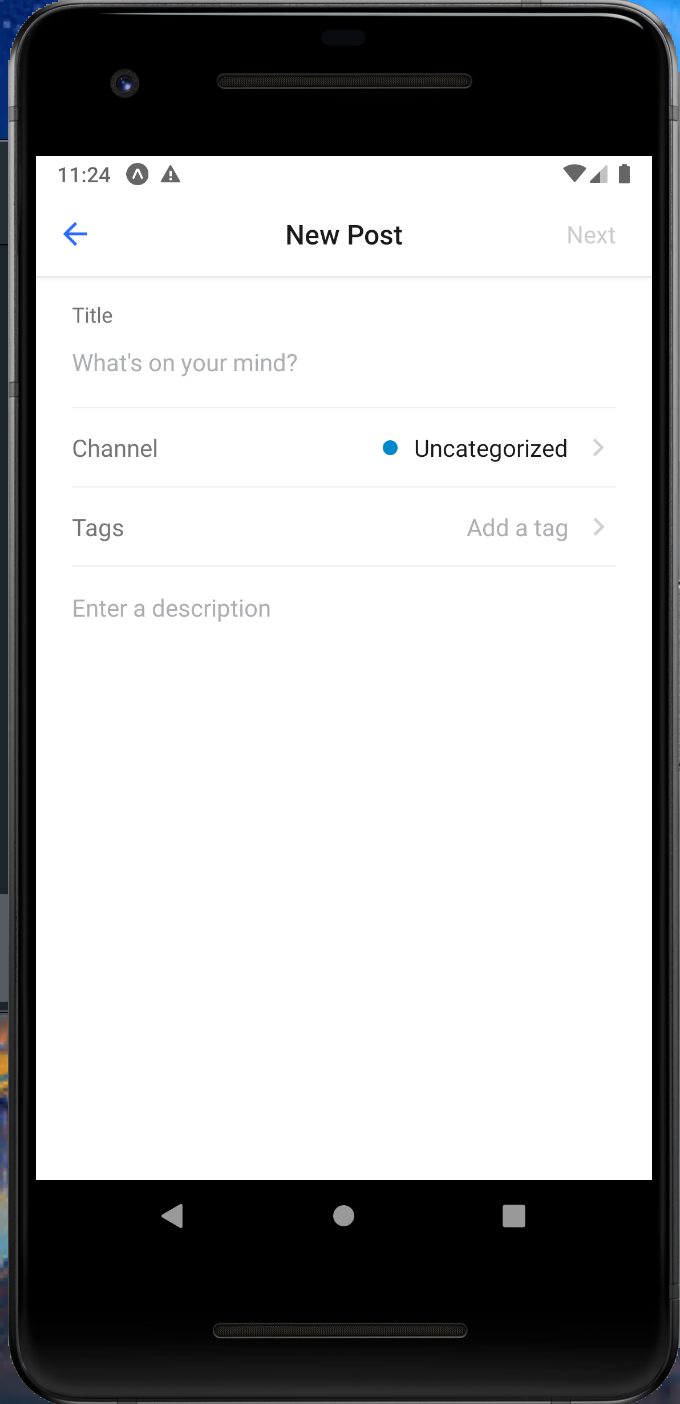The image depicts a mobile interface for creating a new post, which is likely on a smartphone or iPod. At the very top of the screen, numerical indicator '1124' is visible, flanked by various functional icons on both sides. On the right side, there are icons indicating full battery status, internet connection, and phone connectivity.

Centralized near the top is a prominent "New Post" heading. Adjacent to this heading on the right is a "Next" button, while on the left, there's an arrow pointing towards the left, probably indicating a back function. Below this section is a horizontal divider line.

Beneath the line, the first input field prompts with "Title" on the left side and under it, a question "What's on your mind?" indicating where the user can input the title. Another horizontal divider follows this section.

Next, on the left, the label "Channel" is shown, and on the right, the word "Uncategorized" is displayed along with a clickable arrow. A blue dot is positioned just before the word "Uncategorized," which seems to be part of the UI design.

The subsequent section includes a label "Tags" on the left, and on the right is the prompt "Add a tag" with a right-pointing arrow for tag input. 

Following another divider line, the final section on the left has the label "Enter a description," instructing the user to input additional details about their post. The entire UI is set against a clean white background. The layout and design elements strongly suggest that the interface is part of a mobile application, either on a smartphone or an iPod device.